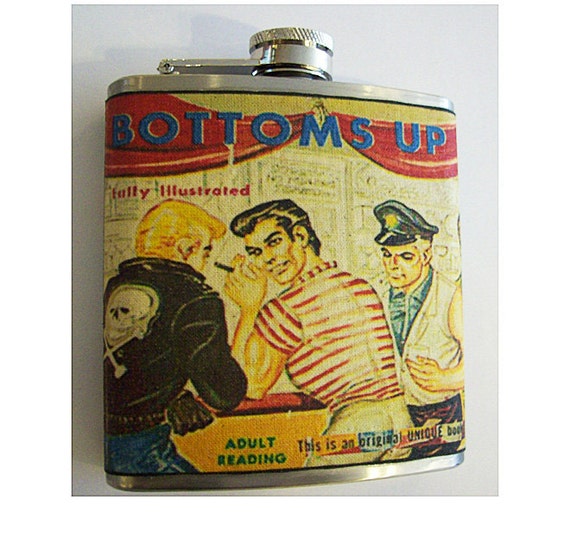This image depicts an antique metallic flask set against a grayish background. The flask features a distinctive silver cap and an illustration wrapped around its body, presenting a vivid and dynamic scene in color. The detailed illustration showcases three distinct characters: 

1. The central figure, standing with his back partially turned, is a muscular man wearing a red and white striped shirt. He has slicked-back black hair and is holding a smoking cigarette.
2. Positioned to his left is a man with slicked-back blonde hair, dressed in a black leather jacket adorned with a white skull and crossbones on the back. This character is also wearing gloves.
3. Behind the man in the striped shirt is a sailor-like figure, donning a sailor hat and a sleeveless white shirt, who appears to be looking down.

At the top of the flask, the words "Bottoms Up" are prominently displayed in blue lettering, followed by "Fully Illustrated." The bottom of the flask reads "Adult Reading." This unique item appears to be an artistically designed flask intended for carrying alcohol, featuring a captivating illustration that evokes a lively bar scene.